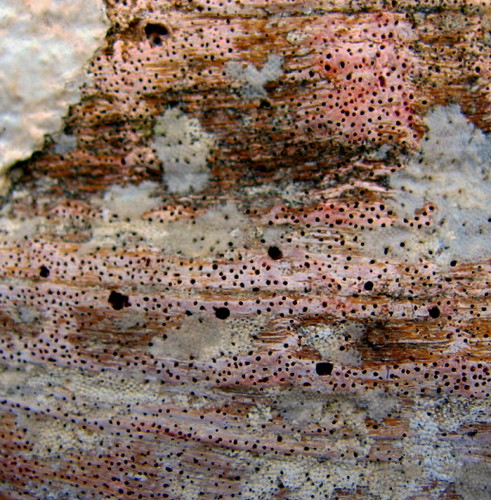The image displays a detailed and intricate surface composed of multiple strips and splotches of white, pink, and red, interspersed with smaller sections of brown. Predominantly, it appears to feature areas resembling quartz, with substantial white and pink sections towards the center and bottom. These sections are accented with numerous black dots of varying sizes, some so dense they form lines running horizontally. Particularly, towards the bottom-left corner, there are small white balls speckled with black, further enhancing the textured appearance. The overall aesthetic is reminiscent of a dessert-like landscape, potentially sitting in white snow, lending an almost surreal, confectionary vibe to the entire scene.